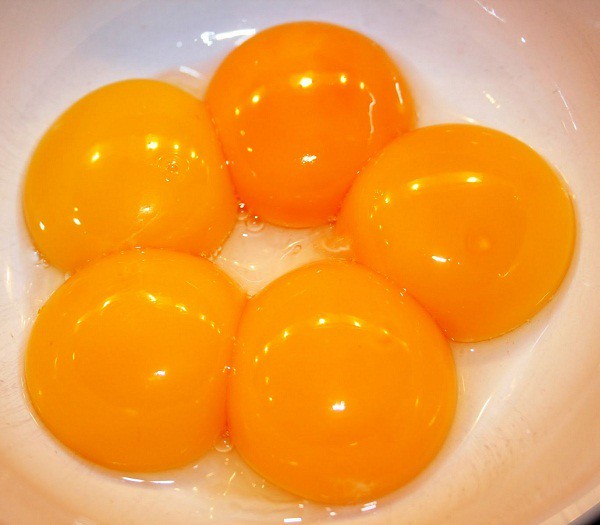In the close-up image, we see five egg yolks arranged in a white bowl, with some egg white visible but mostly focused on the yolks. The yolks are positioned to form a circular, almost flower-like pattern, with a hollow center. The yolk at the top stands out with a darker orange hue compared to the others, which are more of a yellow-orange color. Each yolk, along with the surface of the bowl, reflects dots of light from the overhead lighting, giving them a shiny appearance. The bowl itself is primarily white with a subtle brownish tinge along the edges. Additionally, a small black splotch is noticeable on the right side, suggesting the bowl might be placed on a black table.